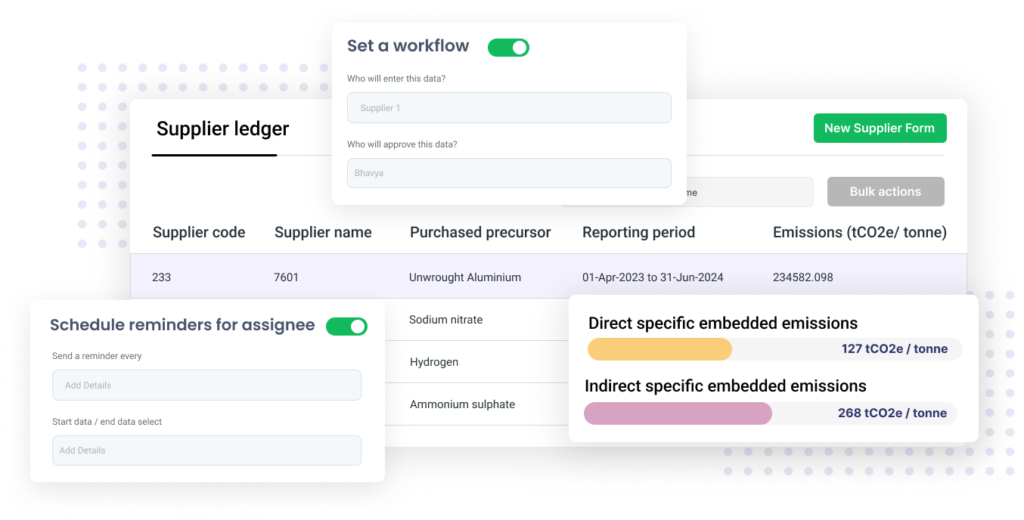The image showcases a digital interface filled with multiple pop-up screens, layered over a white background adorned with gray, rectangle-like dot clusters. The top-left quadrant features a prominent rectangle containing roughly 50 dots, with a smaller cluster situated in the bottom right.

At the center of the interface, a pop-up labeled "Set a Workflow" is visible. This pop-up includes a green toggle button switched to "On." It prompts the user to input "Who will enter data" with a sample entry "Supplier One," and "Who will approve data," shown as "Behavior."

On the bottom left, another pop-up is titled "Schedule Reminders for Assignee," also with the green toggle button set to "On." This section allows for configuring the frequency of reminders with fields labeled "Set a reminder every," "Start Date," "End Date," and "Add Details."

In the bottom right, a pop-up addresses "Direct Specific Embedded Emissions" and displays an orange progress bar that is about one-third complete, indicating 127 tCO2e per ton. Below this, "Indirect Emission Embedded Emissions" are represented by a purple-pink bar, about halfway filled, showing 268 tCO2e per ton.

Beneath these pop-ups, the interface features a section titled "Supplier Ledger" with options to create "New Supplier Form," engage in "Bulk Actions," and fields for "Supplier Code," "Name," "Purchaser Precursor," "Reporting Period," and "Emissions." This portion lists various companies or precursors alongside their respective data.